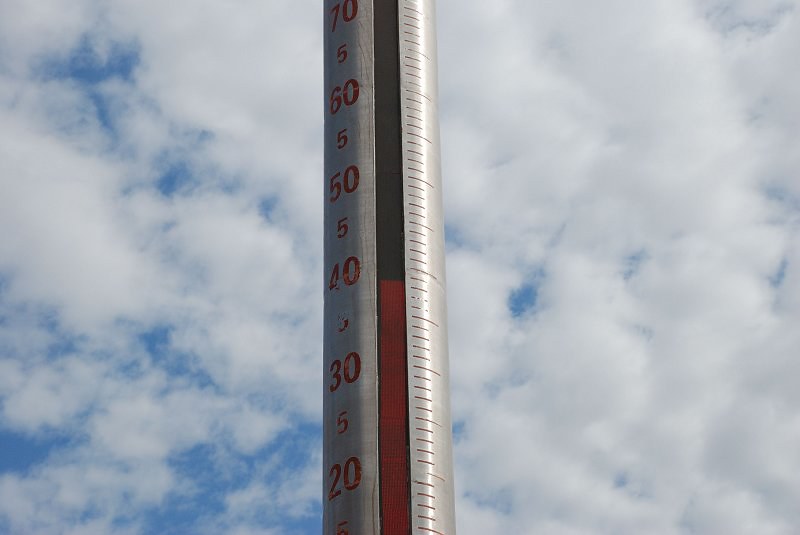The photograph features a predominantly white cloud-filled sky with occasional glimpses of blue, giving the impression of looking directly upward. Centrally positioned, running top to bottom, is a tall, silvery object that resembles a thermometer. Due to the lack of scale, it appears enormous, potentially as tall as a light pole. The object is reflective with a prominent stripe in the center—black on the upper portion and red on the lower.

Both the top and bottom of the object are cropped out of the frame. Clearly visible, red numbers run vertically on one side, starting from 70 at the top, followed by a 5, then 60, another 5, 50, and so on, decreasing in increments of 10 with small 5s in between, suggesting a measurement system descending to zero. The opposite side features corresponding black horizontal marks.

The exact nature of the object is ambiguous, but it appears to be a measuring device, potentially for recording depth or snowfall, given the numerical increments and the context of a snowy environment.